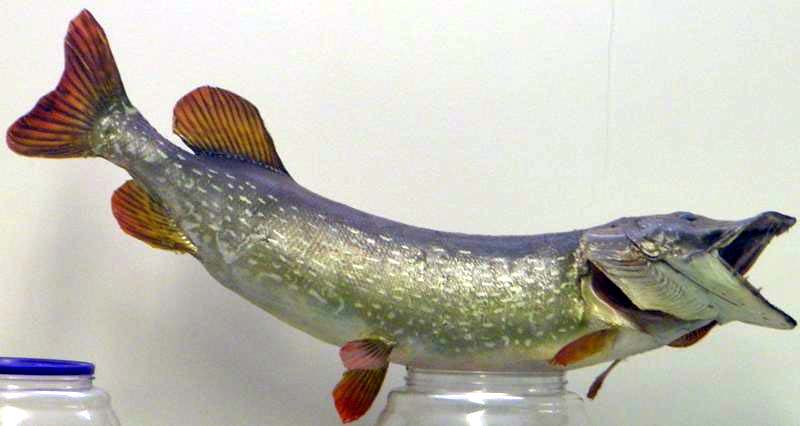In this photo, a fish, possibly a stuffed pike, appears to be resting on the open mouth of a clear glass jar. The fish is a narrow, silver-gray with a tint of green, and features bright orange fins with black streaks. Its mouth is wide open, displaying sharp teeth, and the interior appears dark. The body is stiff and bent in a half-moon shape, with a purplish hue near the top of its back and one visible dark eye. The scene is set against a very white wall, and to the left of the fish is another jar of a similar size with a blue plastic lid. The fish's tail is curved upwards towards the top side of the photo, and overall, it gleams in reflected light, giving it a realistic appearance, resembling a trophy catch.